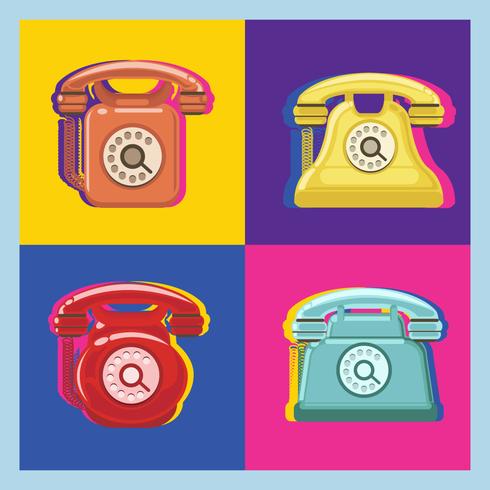This artwork is a vibrant pop art piece reminiscent of Andy Warhol, featuring four distinct rotary phones, each with unique shapes and color schemes. The painting, which has a light blue border, showcases these retro phones arranged in a 2x2 grid. Starting from the top left and moving clockwise:

1. The top-left segment has an orange background with a red rotary phone.
2. The top-right segment features a purple background with a yellow, bell-shaped rotary phone.
3. The bottom-right segment displays a dark blue background with a red, fire alarm-shaped rotary phone.
4. The bottom-left segment shows a fuchsia background with a light blue, robust-base rotary phone.

Each phone includes a white rotary dial that matches the background shade, emphasizing their classic, vintage feel. This colorful, blocked composition makes it a striking poster print suitable for decor in various spaces like bathrooms or living rooms.